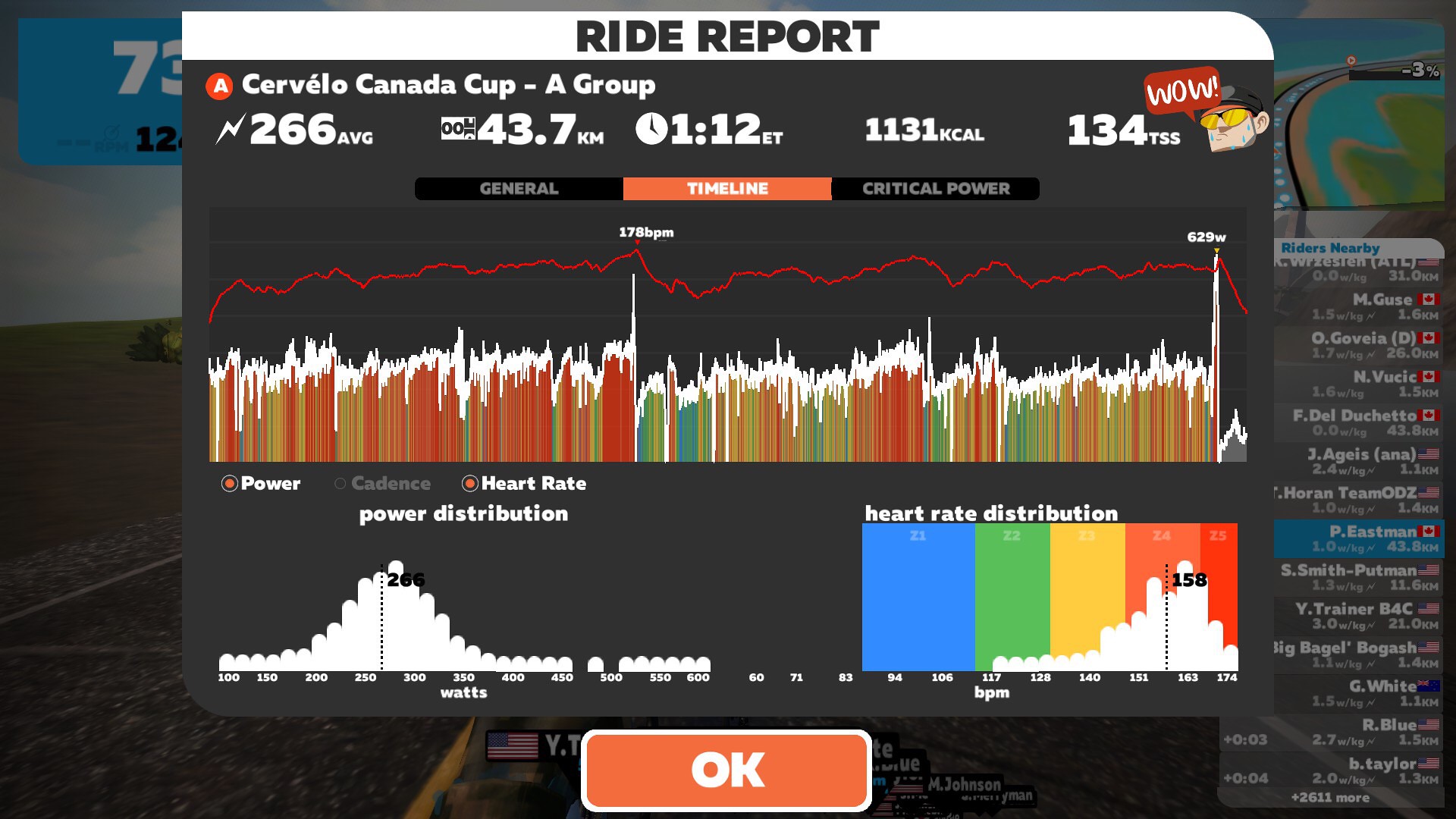The image features a detailed graph set against a black background, showcasing an array of vibrant colors that resemble paint swatches applied with a brush. At the top, "Ride Report" is prominently displayed in black text on a white background. Below, the title "Cervelo Canada Cup" is written in white text, followed by key metrics including "A group," "266 average," "43.7 kilometers," "1 hour and 12 minutes," "ET," "1131 Kcal," and "134 TSS." 

A highlighted tab labeled "Timeline" appears in orange and white lettering, while adjacent tabs labeled "General" and "Critical Power" are in gray. The main graph employs colors like blue, green, yellow, and orange, with a distinctive red trendline overlay. In the lower-left corner, there is a white graph that slopes from small to big and back to small, and on the bottom right, another graph labeled "Heart Distribution" is displayed.